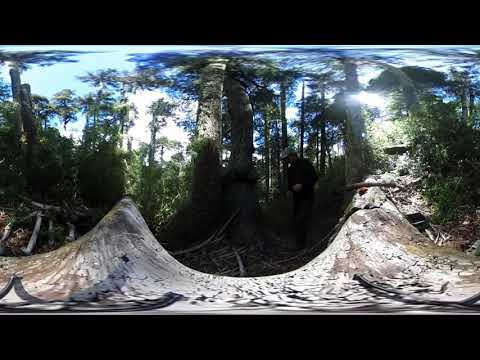This image is a panoramic photograph taken with a 360-degree lens, bordered by black horizontal lines on the top and bottom. The unique perspective distorts the scene, warping the ground on both sides into triangular peaks. At its heart is a densely forested area, likely a rainforest, abundant with tall trees covered in green leaves and vines. The forest floor is littered with downed logs, branches, and sticks, contributing to the intricate texture and clutter below.

In the image's foreground is a prominent tree with gray bark, standing firm among the greenery. Toward the right of the center, a person stands beside this tree. They are wearing a black shirt and dark green pants, and they have a hat, possibly a baseball cap, shading their face. The individual appears to be looking downward. Above the canopy of the trees, a bright blue sky with some clouds suggests that the photo was taken on a sunny day. The overall atmosphere evokes the lush, vibrant essence of a thriving rainforest.